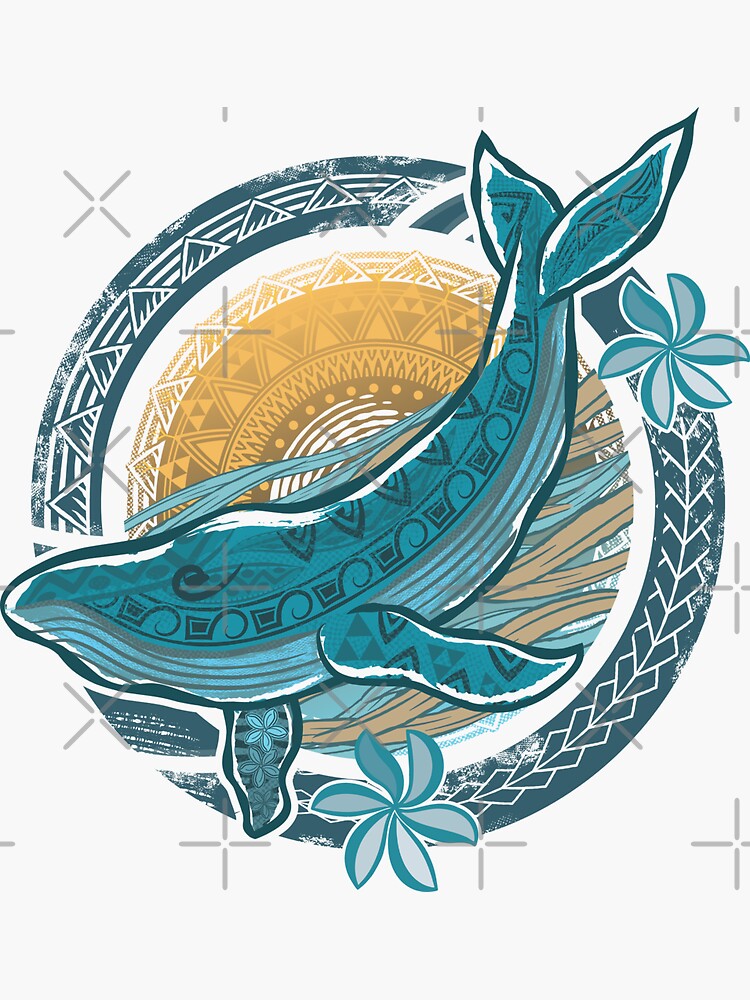The image is a cartoon-style, vertical portrait featuring a prominently displayed blue circle as the background. This circle has a ring of blue gradient around its outer edge. Within this circle, the top left section contains a white three-stripe pattern with equally spaced outward-pointing white triangles. The bottom right section of the circle hosts a single middle line leading to an arrow design pointing in a clockwise direction.

Central to the image is a large, stylized whale, likely a sperm whale, depicted in light aqua blue. The whale's head is oriented to the left, while its tail curves upward to the right. Its body is adorned with intricate spiral patterns and hieroglyphic-like shapes. Covering parts of the circle at approximately the eight o'clock and one o'clock positions, the whale adds a dynamic element to the composition.

Surrounding the whale within the circle are various patterned elements. On the lower right side, there are multiple spirals resembling flowers with leaves, matching the whale's aqua blue color. The upper left of the circle includes blue and brown wavy lines that may represent water.

Additionally, inside the main blue circle, there's another golden circle with a complex design. This inner circle features an outer ring with three stripes and alternating yellow and white triangles. Within this golden circle are several smaller rings with geometric shapes, including dark gray lines and yellow dots.

The image is framed against a white background, enhancing its vibrant blue, gold, and aqua hues while giving a sense of depth and layering to the intricate patterns and whimsical whale design.